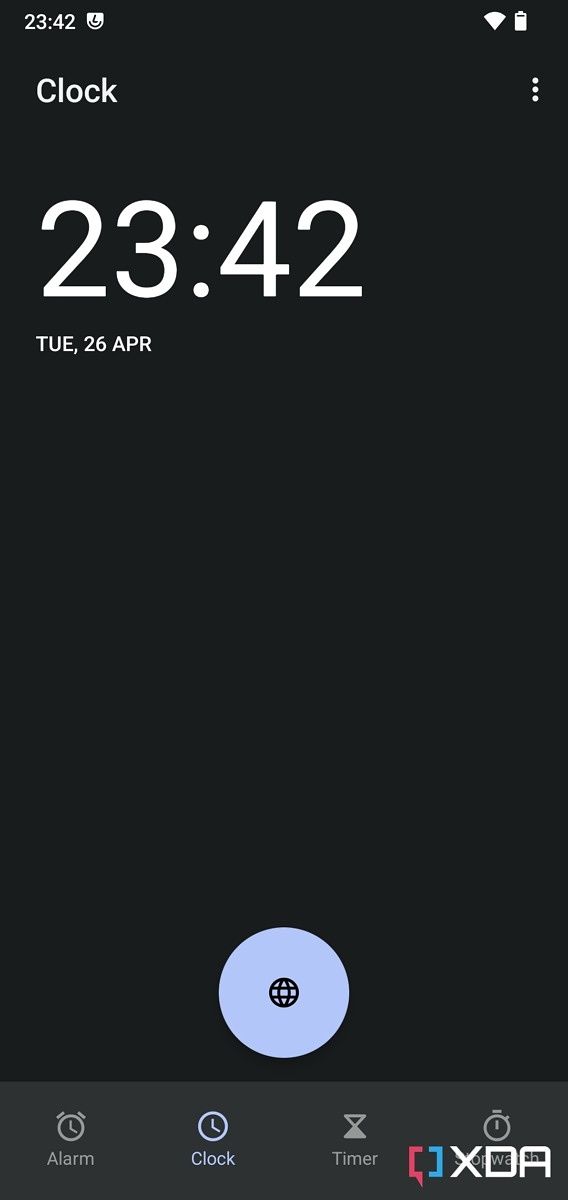Here is a cleaned-up and detailed caption for the described image:

"A screenshot from a smartphone displays a minimalist interface featuring a predominantly black background with white text. At the very top, the status bar indicates the time as 23:42, along with Wi-Fi connectivity and a nearly full battery icon. Directly below, the screen header reads 'Clock' adjacent to a three vertical dots menu icon. The central area prominently shows the large white text '23:42,' with 'Tuesday 26 April' in smaller white text beneath it. The majority of the screen remains blank, emphasizing the simplicity of the display. Near the bottom center, a pale blue circle with a black globe icon adds a subtle touch of color. The bottom of the screen is edged by a dark gray navigation bar resting on the black background, showing icons for Alarm, Clock, Timer, and Stopwatch functions. In the bottom right-hand corner, a distinctive logo features a text box that is half pink and half blue, with the white letters 'XDA' prominently displayed."